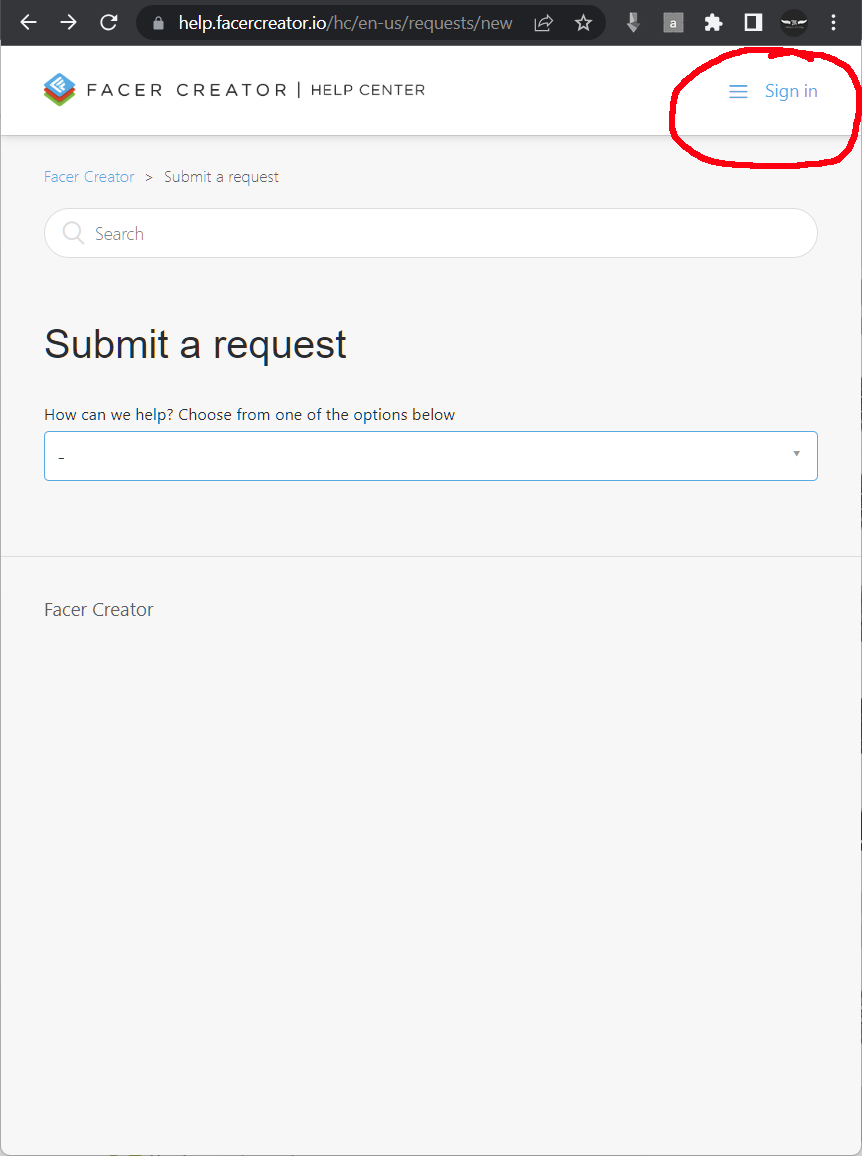A screenshot of the Facer Creator website is shown. The main interface displays three stacked isometric squares in green, red, and blue, with an "F" on the topmost blue square. To the right, the text "Facer Creator" is prominently displayed alongside a "Help Center" link. The URL bar is visible at the top against a dark gray backdrop, featuring various icons related to font downloads, security, and other browser tools.

On the right side of the header, a blue hamburger menu icon is visible, accompanied by the text "Sign In," which has been hand-circled with a red, pixelated pen marking. Below the header, a drop shadow separates the main content area, which begins with another bold "Facer Creator" title followed by the text "Submit a Request."

The central area features a wide search field labeled "Search," which is currently empty. Directly below, large text reads "Submit a Request," with the supplemental text "How can we help? Choose from one of the options below." Beneath this, a drop-down menu is present, but no selections have been made.

A thin line stretches across the full width of the screenshot below the drop-down menu. Further down, the text "Facer Creator" appears again, above a vast, mostly blank rectangular area with only the Facer Creator logo in the upper left. This area has a one-pixel border line on the right edge, distinguishing it from the gray pixel lines elsewhere in the screenshot. Significant darkened sections in the border suggest fragments of an underlying JPEG or image artifact.